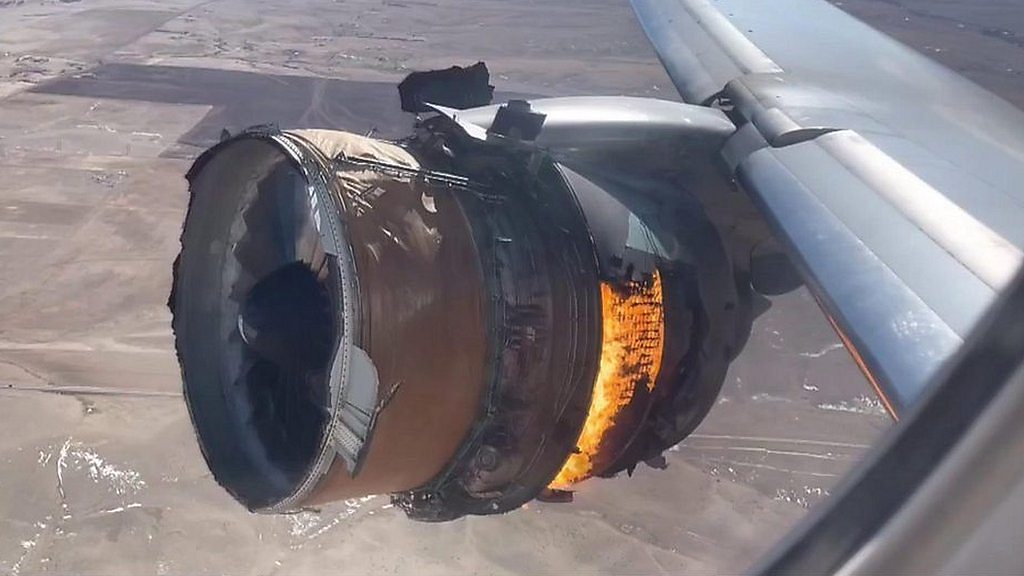This photograph depicts a concerning scene of an aircraft in mid-flight, viewed from a passenger window, focusing on the damaged left wing's jet engine. The engine's exterior appears severely compromised, with the metal casing seemingly ripped off, exposing the internal mechanics. Visible within the exposed engine are uneven and cracked blades, alongside sections where paint is missing. The back section of the engine is particularly alarming, as it shows flames or a glowing fire, indicating active burning. Despite this damage, the wing itself remains undamaged. Beyond the damaged engine, the earth far below reveals a dry, desert-like landscape, emphasizing the high altitude of the flight.